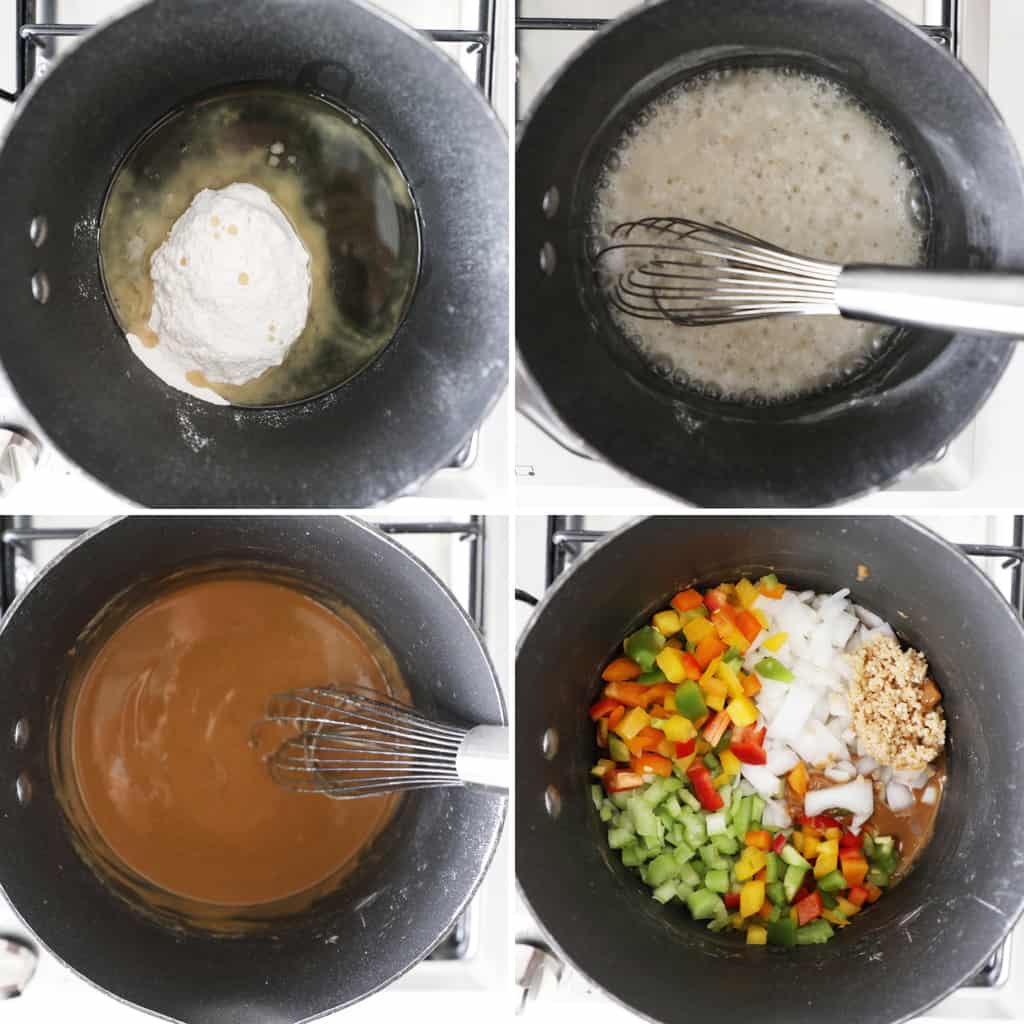The image is a detailed mosaic consisting of four square photographs arranged in two rows, each showing a top view of a dark grey bowl on a cooktop, highlighting different stages of a culinary recipe. In the top left photograph, we see what looks like a pile of white powder, possibly cream cheese, mixed with a liquid, likely cooking oil or water, creating a whitish mixture. Moving to the top right photograph, the mixture is now fully blended, with the entire liquid turning white as it boils and a whisk clearly in use. The bottom left photograph depicts the transformation of this liquid into a rich brown sauce, possibly indicating caramelization or the addition of another ingredient, with the whisk still present. Finally, the bottom right photograph showcases an array of colorful, finely chopped vegetables, including bell peppers in green, yellow, and red, along with onions and possibly celery stalks, mixed into the brown sauce, with an additional element that resembles brown sugar or panko sprinkled on top. This series of images comprehensively illustrates the progression of preparing a dish from initial ingredients through intermediate stages to the final mix of vibrant vegetables and sauce.